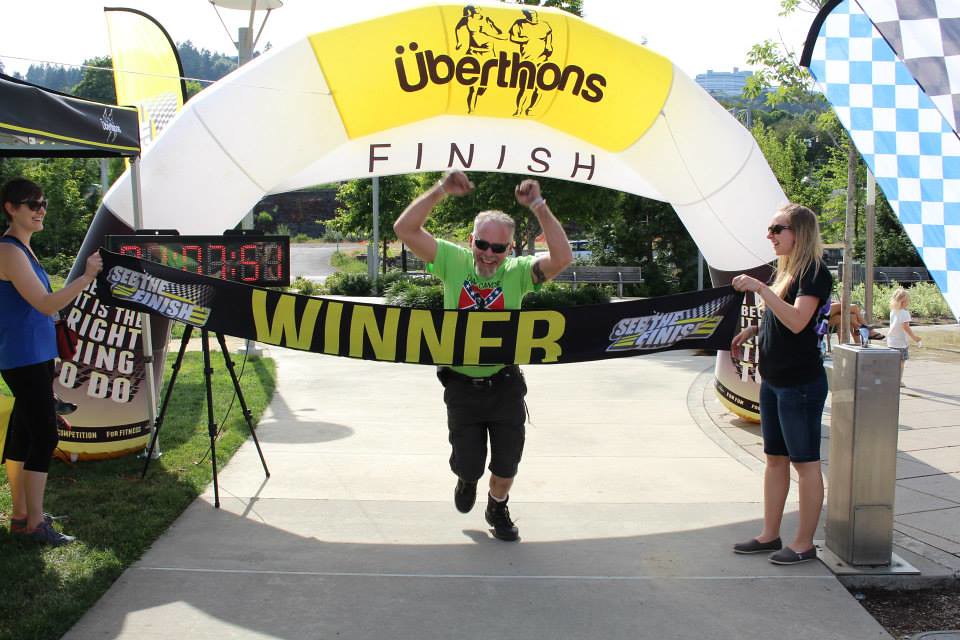This image captures a marathon race called Uber-thons, set in a scenic park environment. In the foreground, an older gentleman is triumphantly crossing the finish line, both arms raised high, his face adorned with a wide smile and sunglasses. He wears a standout lime green shirt featuring a red confederate flag in the center, black pants, and boots. As he crosses the finish line, he breaks through a black banner with the word "Winner" emblazoned in yellow, held on either side by two Caucasian women. Above him, an inflatable arch bears the "Uber-thons Finish" insignia, with an adjacent clock documenting the race time. The background reveals leafy green trees, shrubbery, and a wandering child to the right, adding life to the lively park setting. A blue and white Bavarian flag decorates the right side, while on the left, a domed tent and a simpler, flat-roofed tent are visible, alongside a statement reading "It is the right thing to do" under the Uber-thons signage. This vibrant snapshot embodies the spirit and setting of the Uber-thons marathon.